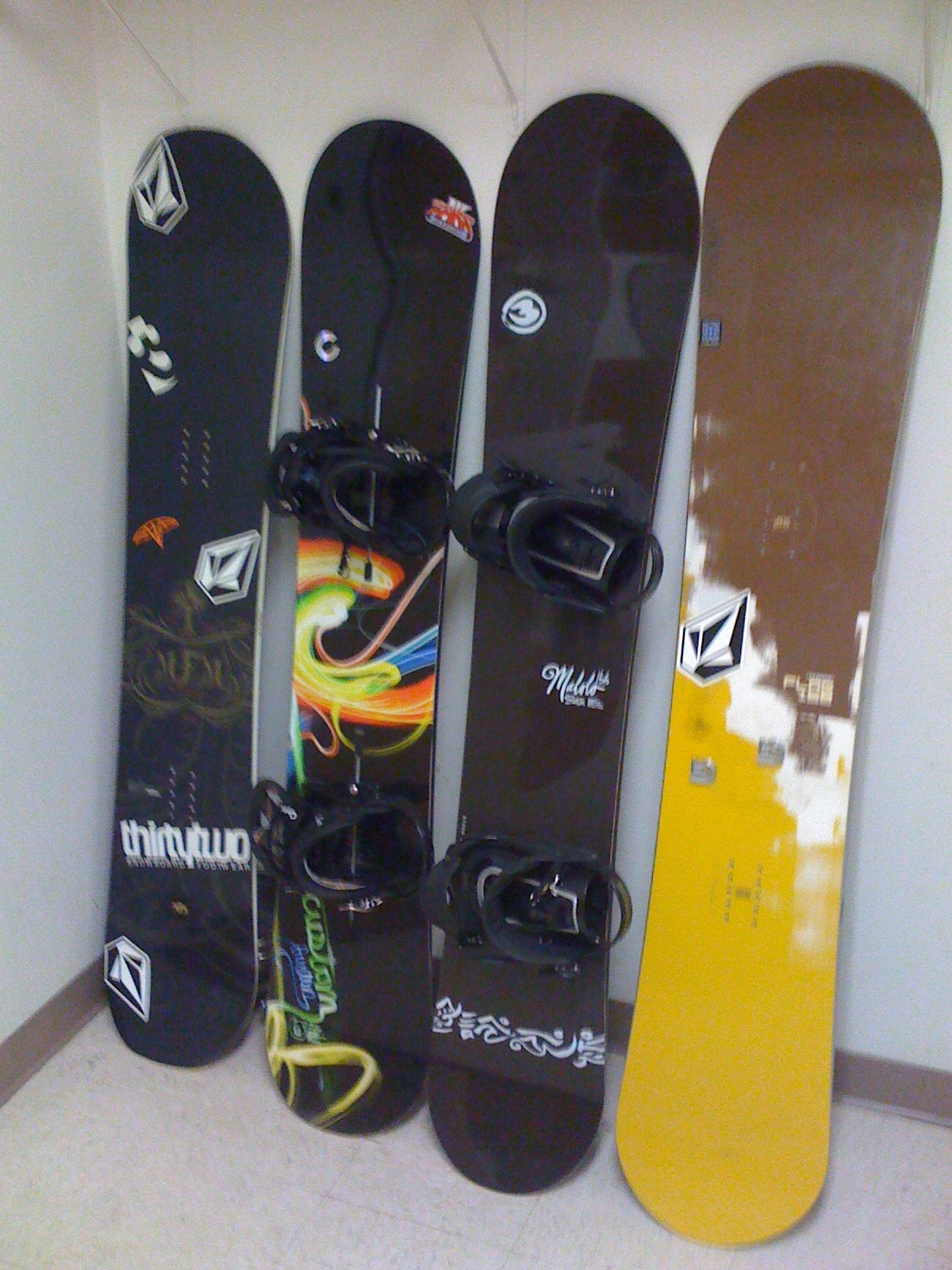This vertical, realistic photograph, set indoors, shows four snowboards leaning against a slightly off-white to light-blue wall with a small section of the left wall also visible. The walls feature a brown trim that runs about four inches high, and the floor is covered with beige linoleum tiles. Each snowboard is distinct in design: 

1. The leftmost snowboard is black with white symbols and the text "32" in bold, lacking bindings.
2. The second snowboard is black with black bindings, adorned with red and green swirly designs.
3. The third, also black, has black bindings with white text and designs that are difficult to decipher.
4. The rightmost snowboard has no bindings, featuring a brown top, a mustard yellow bottom, and a white cloud-like design separating the two colors.

The snowboards appear well-used and are positioned side by side with narrow strips of the wall visible between them. The scene includes other minor details such as small gray spokes protruding from the wall at the top, which remain unclear in their function. The overall atmosphere suggests a storage room or corner of a house, familiar yet functional.